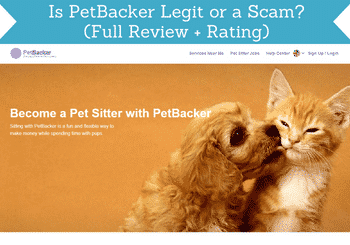The web landing page features an engaging design, starting with a prominent banner that spans the entire top portion of the page. The banner boasts a light blue background adorned with white, inward-pointing triangles, creating a ribbon-like aesthetic. At the center, bold white text reads: "Is Pet Backer Legit or a Scam?" followed by a subheading in parentheses: "(Full Review plus Rating)."

Below the banner is a straightforward navigation header with a white background. To the left, the Pet Backer logo is displayed prominently next to the site's name. The navigation bar includes four blurry, clickable tabs. The third tab features a circular icon with a dropdown menu, while the fourth tab is marked "Sign Up/Log In."

The main section of the page has a vibrant orange background, showcasing an adorable young puppy on the left and a kitten on the right. The puppy is playfully turning its head and licking towards the kitten's mouth, while the kitten squints its eyes in a charming expression. Both animals have orangish-yellow fur, with the kitten sporting a bit of white fur on its belly. Notably, the kitten's ears stand upright, while the puppy's ears droop down.

At the upper left of this section, white text reads: "Become a Pet Sitter with Pet Backer." Beneath this headline are two lines of smaller text in white font: "Sitting with Pet Backer is a fun and enjoyable way to..." The remainder of the second line is too blurred to read clearly.